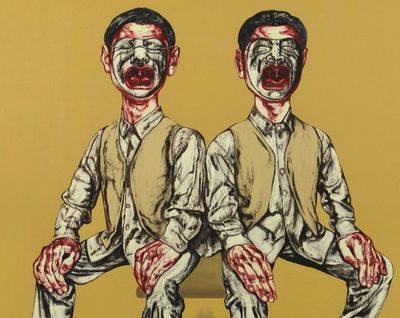The image is a square caricature drawing of two men or boys, both of whom are Caucasian. They are seated closely together on a single yellow stool against a mustard brown background. Both figures have exaggeratedly large hands, which are noticeably red and appear bloodied, resting on their knees. Their heads and necks share the same crimson hue, creating a vivid and unsettling contrast. Each figure has short brown hair and closed eyes with white paint covering their eyes, nose, and mouth, intensifying the eerie atmosphere. They are both wearing long-sleeve button-down shirts and matching mustard-colored vests, paired with greenish-tan pants. Their mouths are agape, as if in a scream, revealing the insides of their throats and even their tonsils, further adding to the disturbing nature of the scene.